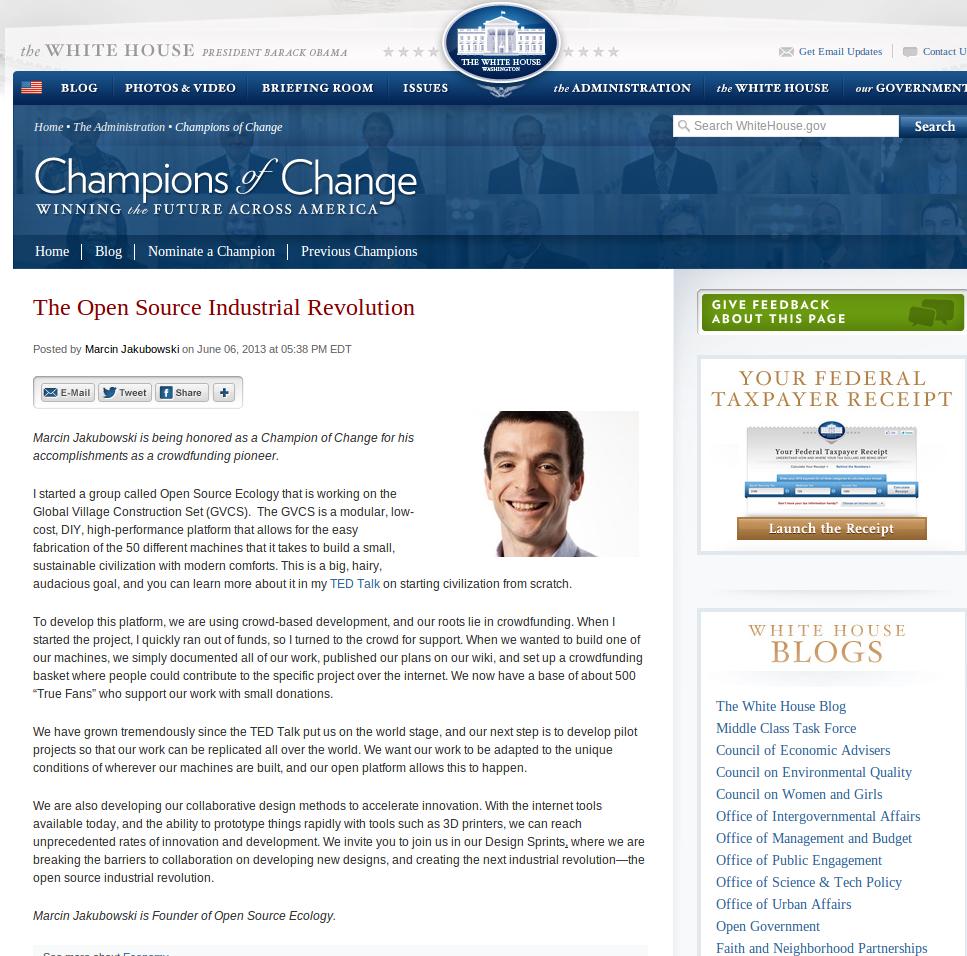A detailed view of an article on the official White House website during President Barack Obama's administration. The article, titled "The Open Source Industrial Revolution," is authored by Marcin Jakubowski. It details the work of Open Source Ecology, a group Jakubowski founded to develop an open-source platform utilizing crowd-based development and funding. The page is minimalist, with a clean white background and a blue top banner. The navigation bar at the top includes links to "Blog," "Photos and Video," "Briefing Room," "Issues," "The Administration," and a "Contact Us" button. The right pane features links to other White House blogs, but there are no pictures of President Obama. The interface is straightforward, focusing on content rather than imagery.